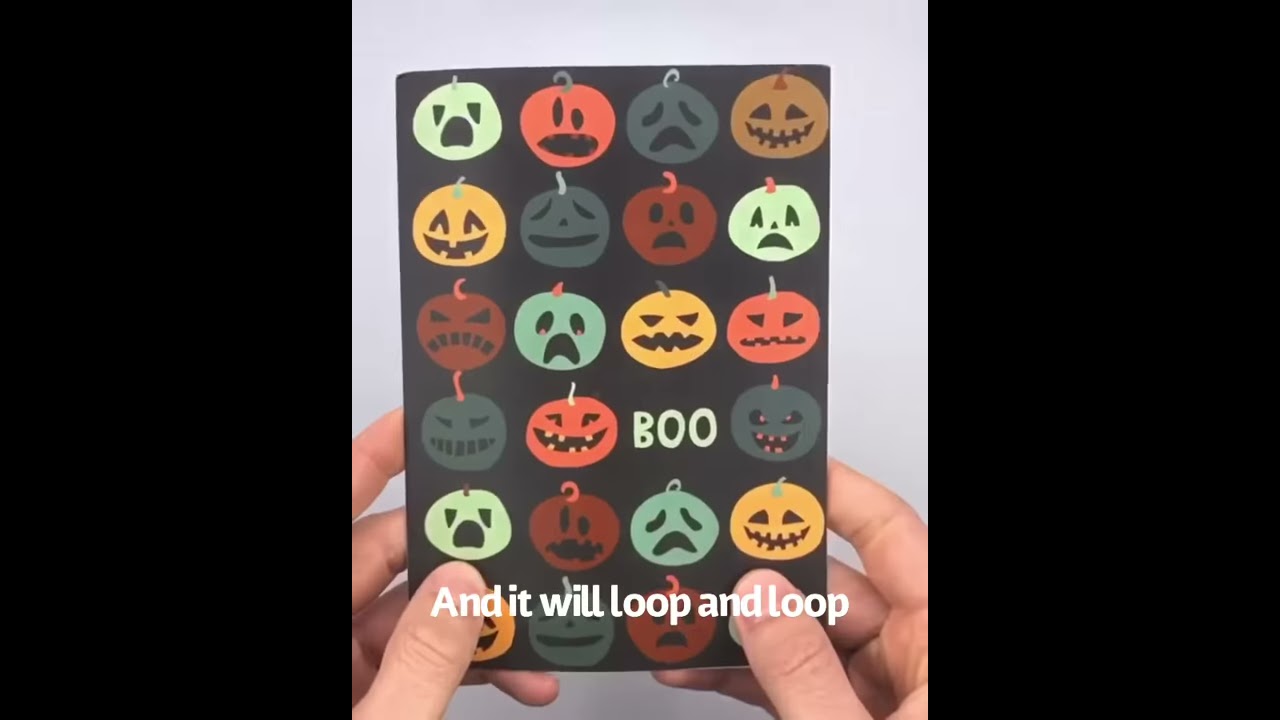In this wide rectangular image, two hands with white skin hold a Halloween card against a light blue or gray background. The hands are positioned near the bottom of the frame with thumbs pressed against the card's lower sides and fingers behind it. The card itself is predominantly black and features a row of variously colored jack-o'-lanterns, including white, red, black, brown, yellow, and orange pumpkins. Each pumpkin sports a different facial expression, ranging from happy to menacing and even ghostly. In the center of the card, "boo" is written in white font. The image is framed by thick black rectangles on either side, and at the bottom of the image, white text reads, "and it will loop and loop." The backdrop is a plain white wall.